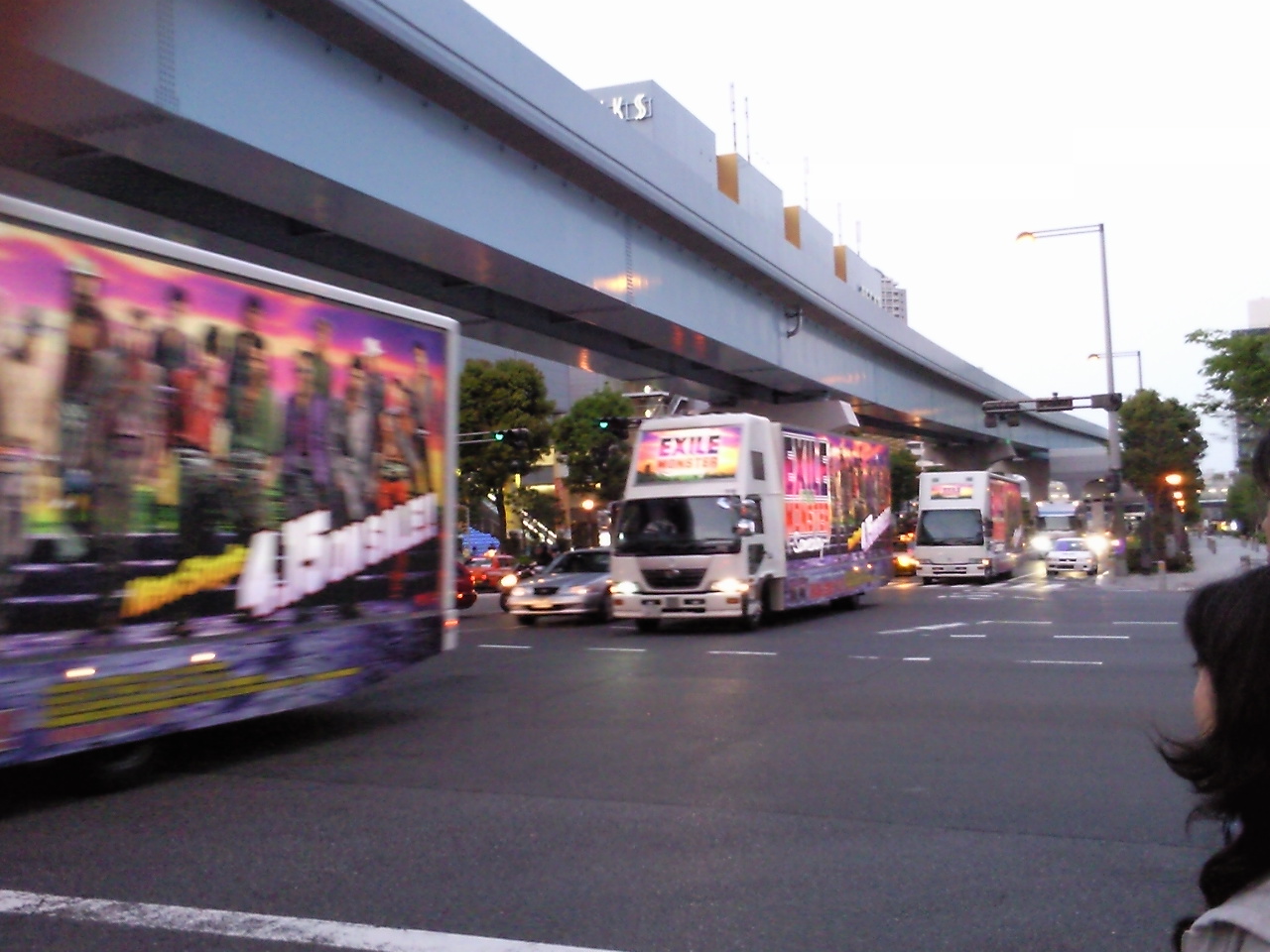This outdoor landscape photograph, despite its low resolution and slight blur, captures a bustling intersection where multiple colorful trucks are moving towards the camera from the left-hand side at a diagonal. The grainy image reveals vibrant trucks decorated with imagery and text, although motion blur obscures some details. Notably, a truck in the center features the words "Exile Monster" prominently on its front and side. Above the traffic is a reflective, shiny bridge made of grey marble, but its purpose remains unclear as no activity is visible on it. Headlights of several vehicles suggest the scene is either early morning or late at night, under an overexposed, featureless white sky. In the background, there are taller buildings and street signs, with patches of trees visible on both sides. In the bottom right corner, the partial figure of a woman with dark black hair is captured, further illustrating the everyday hustle of this busy urban setting.